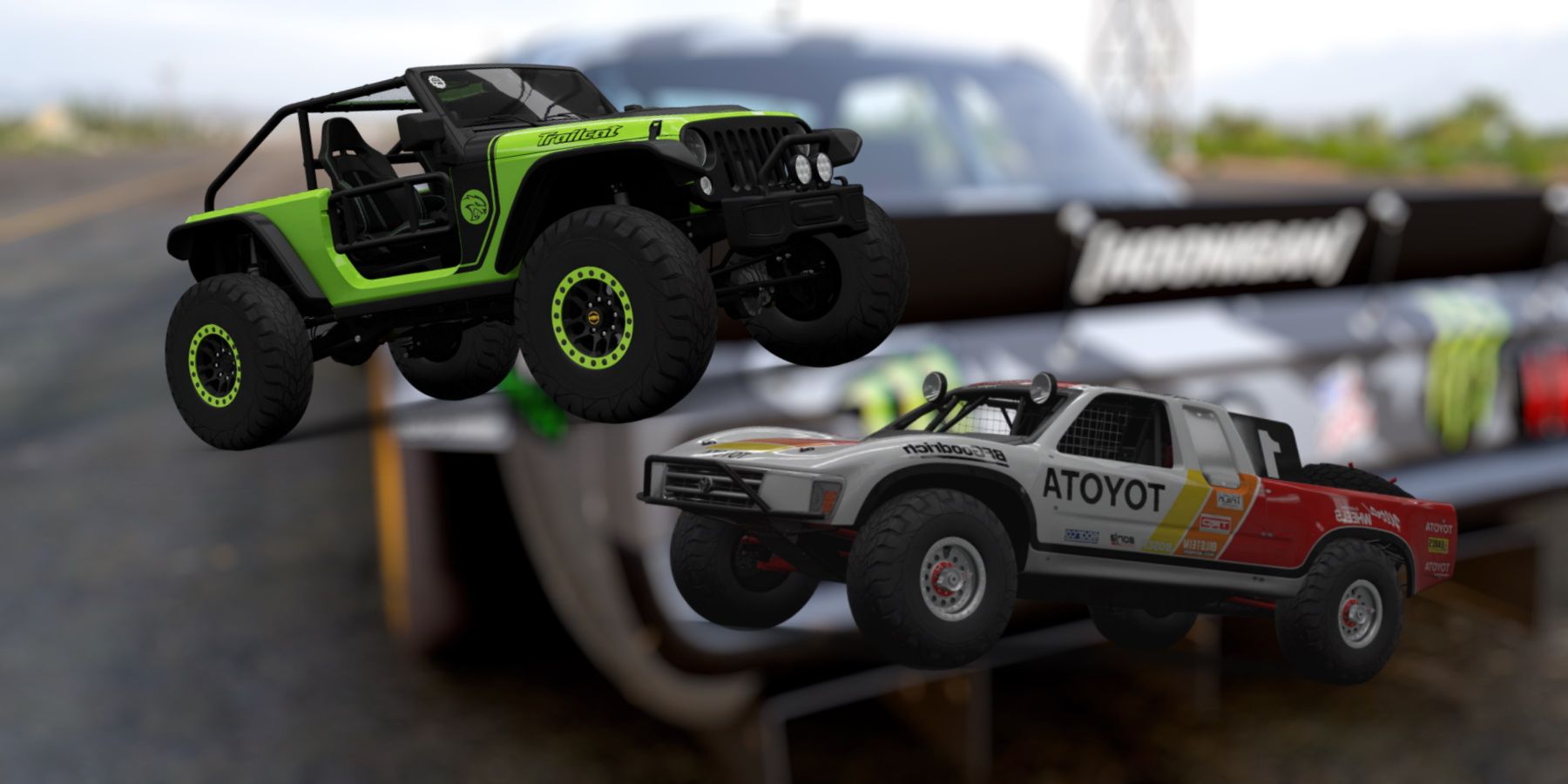The image depicts two distinctive racing vehicles prominently positioned against a blurred background. The first vehicle, located on the left, is a vivid lime green, open-top Jeep. This Jeep features massive black tires with lime green rims, a roll bar instead of a roof, and black seats secured with additional metal bars. Notable elements include its large, independently standing windshield at the front and its overall rugged, off-road design.

The second vehicle, positioned to the right, is a pickup truck with oversized tires and bold, eye-catching colors. The truck's body is primarily gray, accented with stripes of red, orange, and yellow on the rear fender, hood, and roof. The truck displays the word "ATOYOT" backwards, likely indicating it is a Toyota. It also features large fog lights or headlights above the regular ones, a grill guard, and a roll cage. 

In the background, an out-of-focus car with yellow-rimmed wheels faces away from the camera, with some trees barely visible, adding depth to the scene. The overall composition highlights both vehicles' robust and sporty designs.